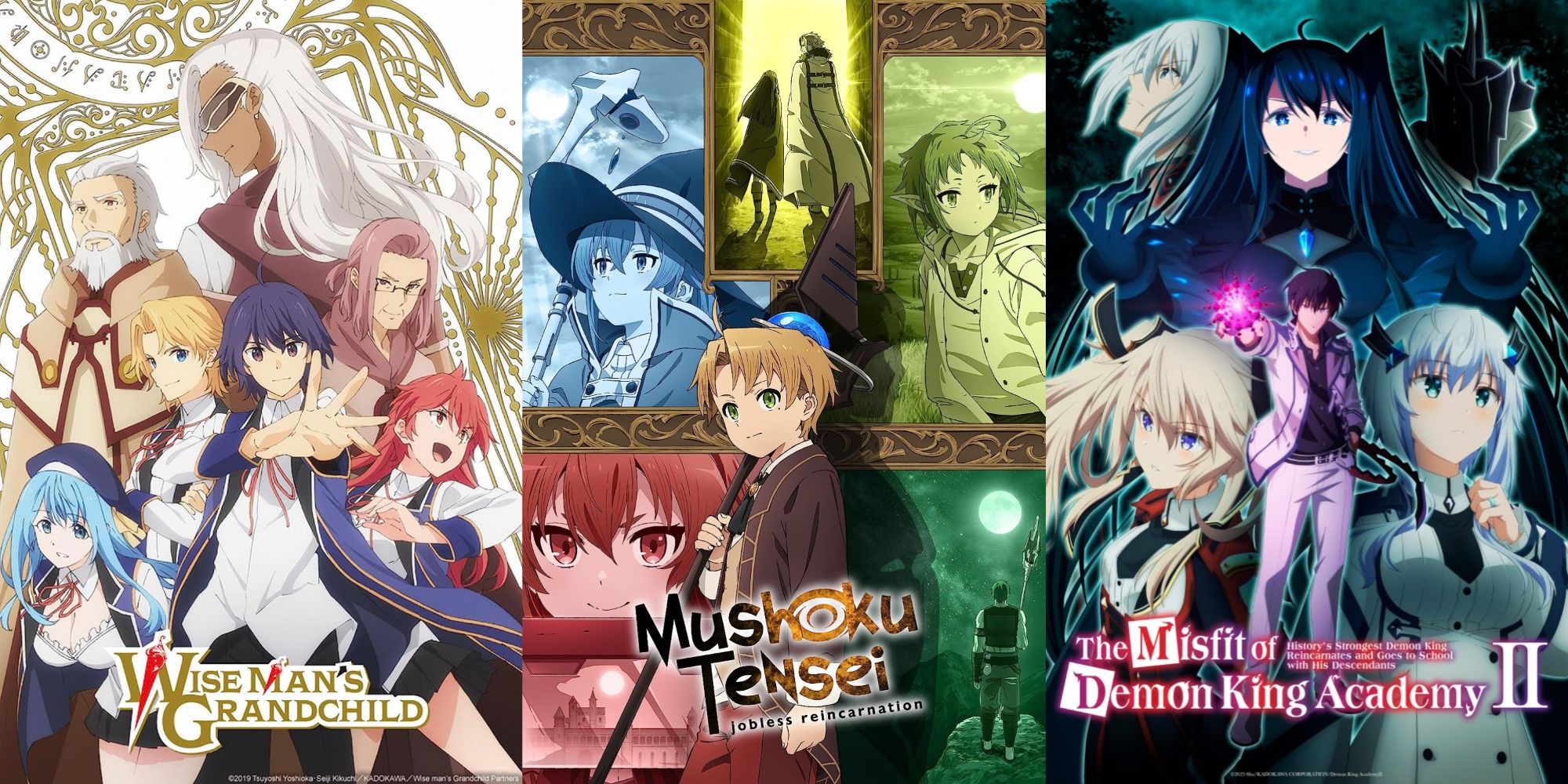This is a horizontal image displaying three colorful anime posters, each representing a different show. The leftmost poster is titled "Wise Man's Grandchild." It features a blue-haired boy wearing a blue cloak, a white shirt, and black pants, extending his left arm outwards. Surrounding him are vibrant characters, including a busty blue-haired girl to his left, a red-haired girl, a blonde girl, an old man with pink hair, an old blind man with white hair, and another elderly man with a beard. The middle poster is titled "Mushoku Tensei, Jobless Reincarnation," depicting a young boy with brown hair holding a stick, seemingly a flagpole. Behind him are various background characters, including witches. The rightmost poster is for "The Misfit of Demon King Academy II." It centers on a man in a white suit and black shirt, extending his right arm while holding a glowing purple ball. Surrounding him are three striking female characters with different hair colors: white, blonde, and black.